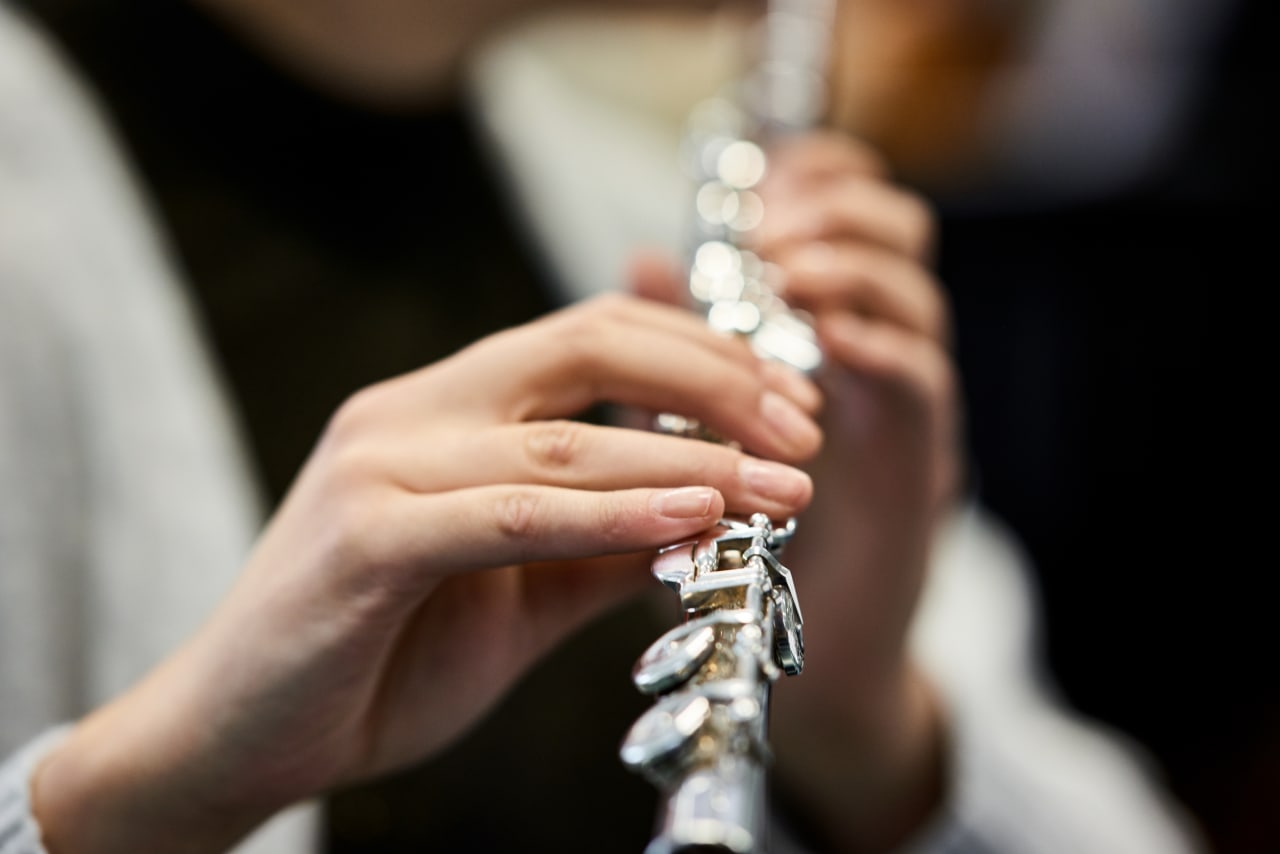This detailed close-up photograph captures a silver flute being played by a person with youthful, light-colored hands. The image is sharply focused on the left hand, which is engaged in pressing the flute's keys, while the right hand remains blurred in the background, resting on the upper portion of the instrument. The person, who appears to be wearing a white cardigan-style sweater over a black shirt, has short, non-manicured nails. The background is heavily blurred, displaying a mix of black, brown, and blue hues, with the right side of the picture particularly out of focus. The rectangular-shaped image does not reveal the person's face or the part of the flute being blown into, maintaining the primary focus on the interplay between the hands and the instrument.